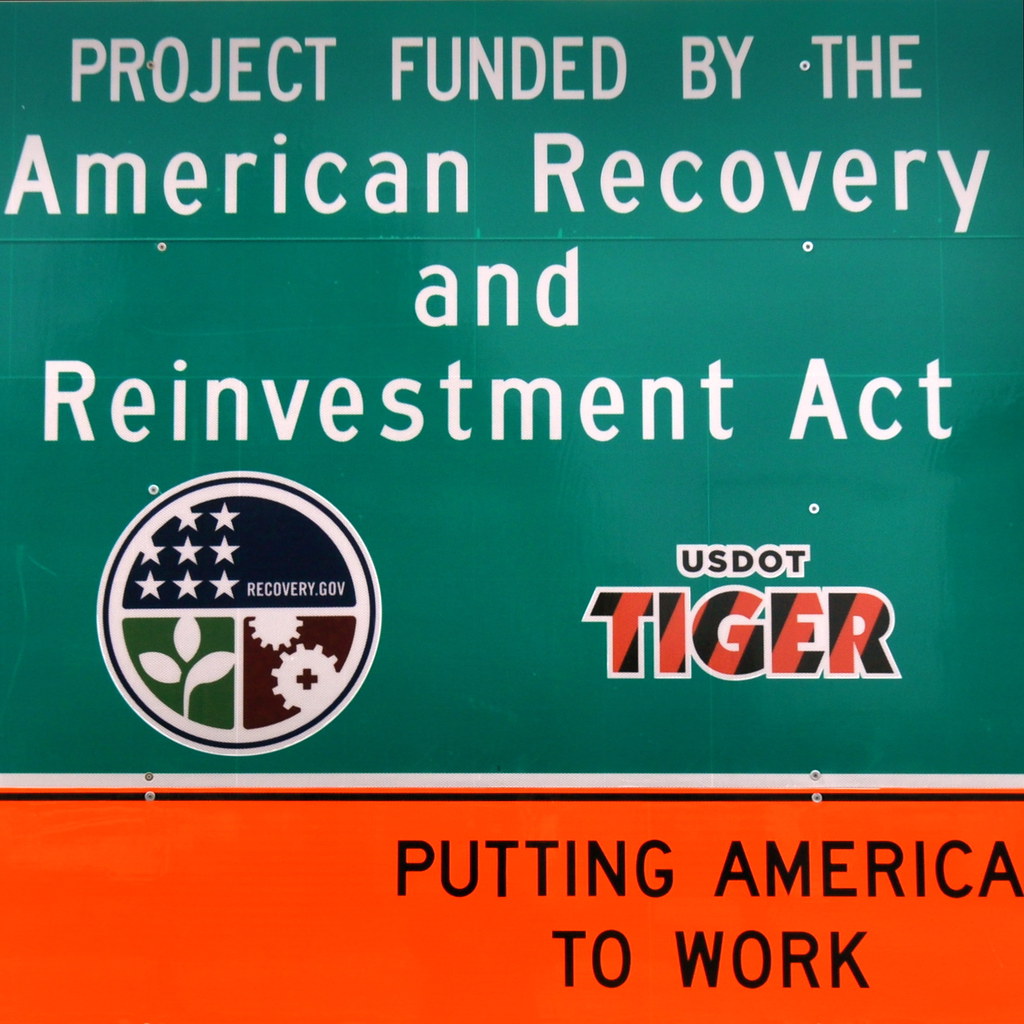The image features a public service announcement sign with a predominantly two-toned color scheme, divided into a larger top portion in green and a bottom portion in orange. The top portion is topped by white, capitalized, sans-serif text that reads "Project Funded by the American Recovery and Reinvestment Act." Below this white text is a pair of logos. The left logo is a white circle with a black border. The upper half of the circle contains a blue semi-circle with white stars, and the phrase "Recovery.gov." The lower half of the circle is divided into two quadrants: a green section with a white trifoliate branch and a brown section with white gear graphics. To the right of this logo is another logo with the text "US DOT" prominently outlined in white, followed by the word "Tiger" in bold, orange, and black diagonal stripes, also outlined in white. A thick white horizontal line and a thinner black line separate the top section from the bottom, which is orange. Centered within the orange section, in black text, are the words "Putting America to Work."